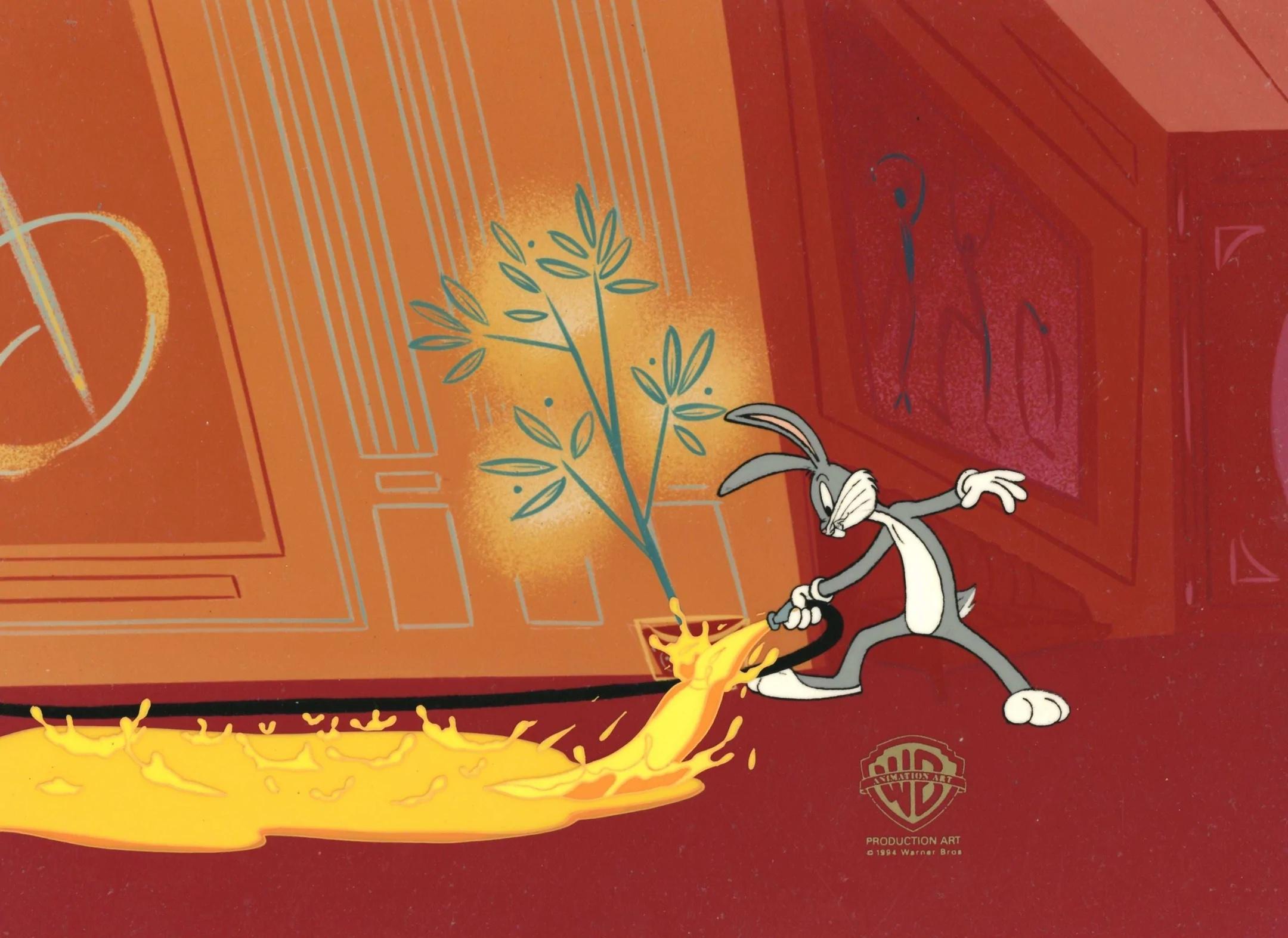This detailed caption combines the information from all three sources:

The image is a screenshot from a Warner Bros. Bugs Bunny cartoon. It depicts Bugs Bunny, the iconic gray rabbit with a white stomach, gloves, paws, and mouth, along with his signature long gray ears with pink inner sections. Bugs Bunny is in a long red hallway, with a red carpet and orange walls adorned with line art decorations. He is pulling a black hose from the left towards the right, and from the hose spills a yellow, sticky-looking substance that is splashing onto the floor. Bugs Bunny appears to be setting up some sort of trap or prank, as he walks towards the right with a focused expression. A potted plant stands directly behind him. Below him, there is a watermark that reads "WB Production Art," subtly blending into the red carpet.